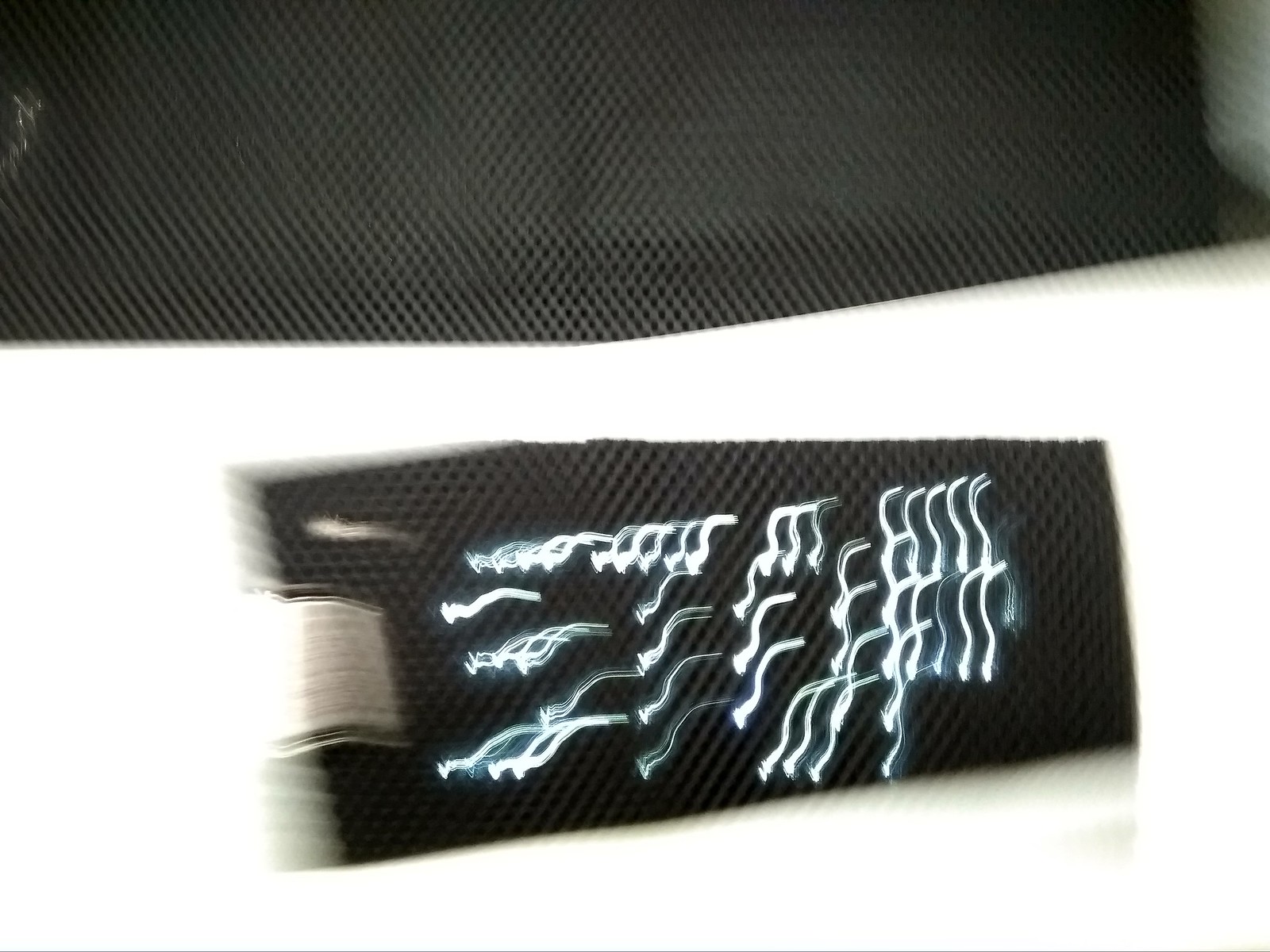On a white square background, the image features a horizontally oriented, nearly rectangular section in the upper portion, adorned with gray fabric. The fabric, which has a slightly thicker depth, is decorated with a pattern of minute crosses forming small diamond shapes. Below this section, there is a cut-out piece of the fabric, with a small white flap on the right side. Superimposed on the fabric, seemingly computer-generated, are white squiggly lines resembling thin 'S' shapes. These squiggles form a grid-like pattern consisting of approximately four columns down and four to five rows across, depending on the specific area you're observing.